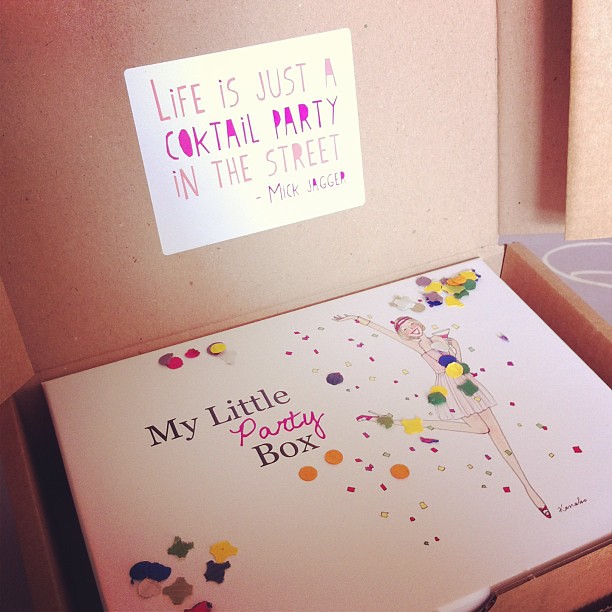The photograph depicts an open cardboard box with its lid propped up, revealing a sign on the interior of the lid that reads, "Life is Just a Cocktail Party in the Street" by Mick Jagger, though "cocktail" is misspelled as "coktail." Inside the box is another white box labeled "My Little Party Box," with "party" highlighted in pink and the rest in black typed letters. The white box features a cartoon drawing of a ballerina-like lady wearing a short white dress, pink high heels, and a pink cap or bandana. Her right hand is raised as if she's dancing, and her right leg is playfully flipped back. She holds a champagne glass in her left hand. Surrounding her are colorful confetti and celebratory decorations, giving the entire scene a festive, party-like atmosphere.